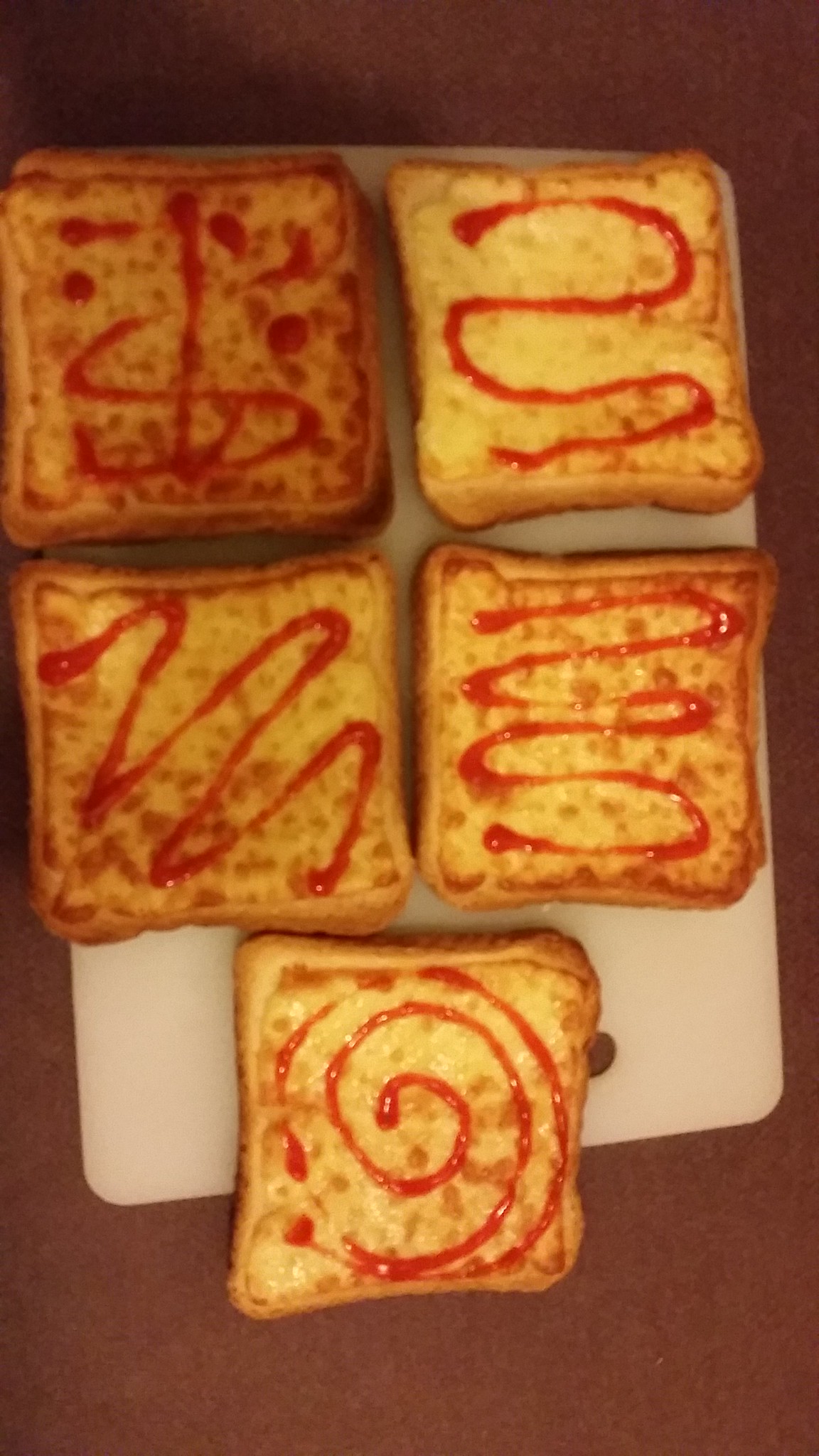This detailed photograph provides a close-up view of a dark brown and reddish wooden tabletop or counter. Centrally positioned on this surface is a rectangular white plastic cutting board, oriented vertically. Arranged on the cutting board are five golden-brown grilled cheese sandwiches, accented with buttery and seared textures. Each sandwich is artfully adorned with a drizzle of red sauce, possibly ketchup or hot sauce, creating a variety of patterns. The sandwiches are organized in a two-two-one formation: two at the top, two in the middle, and one at the bottom. The drizzled sauce on each sandwich forms unique shapes, ranging from swirls and zigzags to almost circular patterns, adding a whimsical touch to the cheese-laden tableau.